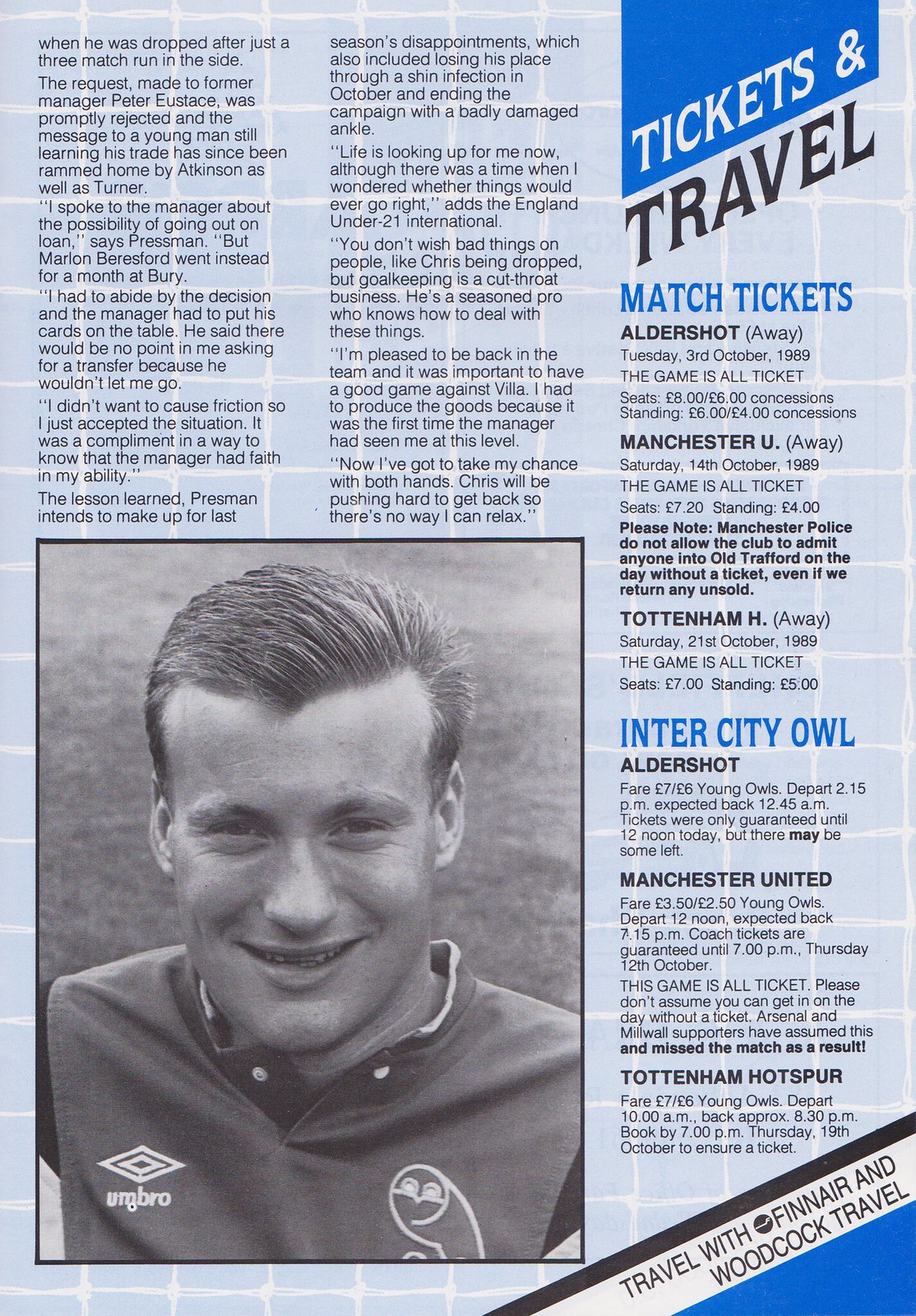The image depicts a page from a magazine or newspaper, featuring a structured layout with an emphasis on football match information and a player interview. The background is light blue with white horizontal and vertical stripes, creating a defined grid-like appearance.

In the top right corner, there's a blue trapezoid with the text "TICKETS AND TRAVEL" in bold black letters, and directly below it, two headings: "MATCH TICKETS" and "INTERCITY OWL." Detailed ticketing information follows for various matches:

- **Aldershot Away:** Tuesday, 3rd October 1989. This game is all-ticket with seating priced at £8 (€8) or £6 (€6) with concessions, and standing tickets at £6 (€6) or £4 (€4) with concessions.
- **Manchester United Away:** Saturday, 14th October 1989. The game is all-ticket with seats at £7 (€7) and standing at £4 (€4). Note that Manchester Police will not admit anyone without a pre-purchased ticket.
- **Tottenham Hotspur Away:** Saturday, 21st October 1989. The game is all-ticket with seats at £7 (€7) and standing tickets at £5 (€5).

Additional travel information is featured for supporters, including fares and departure details for each match through the "Intercity Owl" service.

On the bottom left is a black-and-white photograph of a smiling football player with medium-length hair, accompanied by an extensive article detailing his experiences and career challenges. The text describes his interactions with management, highlighting a specific incident involving former manager Peter Eustace, and provides insights into his journey through injuries and professional setbacks. The player expresses a determined outlook on his future in the sport.

Towards the bottom right, the page also mentions "Travel with Finnair and Woodcock Travel" in a blue triangle, further emphasizing travel arrangements for supporters.

This comprehensive layout provides readers with detailed information on upcoming matches, ticketing, and travel arrangements, enriched by a personal narrative from a featured player.